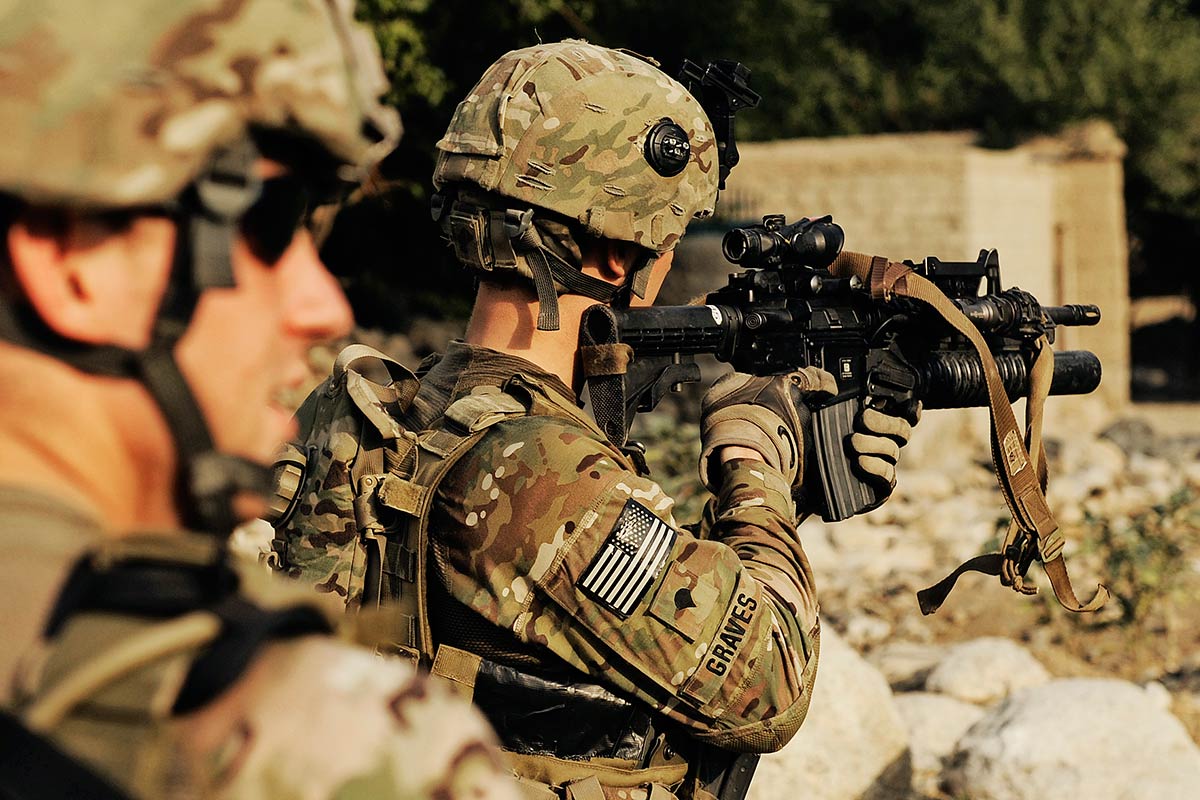This detailed close-up photograph captures two military personnel, likely from the U.S. Army, amidst a training exercise or combat scenario. Both individuals are dressed in full camouflage gear, including helmets and backpacks. The person on the left is closer to the camera and out of focus, partially visible up to their shoulder, and appears to be male, looking off to the right side of the image. Although their face is obscured, they are wearing sunglasses and a helmet.

The main focus of the image is the second individual, slightly behind the first. This person is in sharper focus and is seen from behind, holding up a machine gun. The back of their helmeted head is in view, and they are sporting gloves and a backpack. A patch on their right arm displays the name "Graves" along with an American flag. The background reveals a mix of greenery, rocky terrain, and a sandstone-like structure, suggesting a rugged training or combat environment.